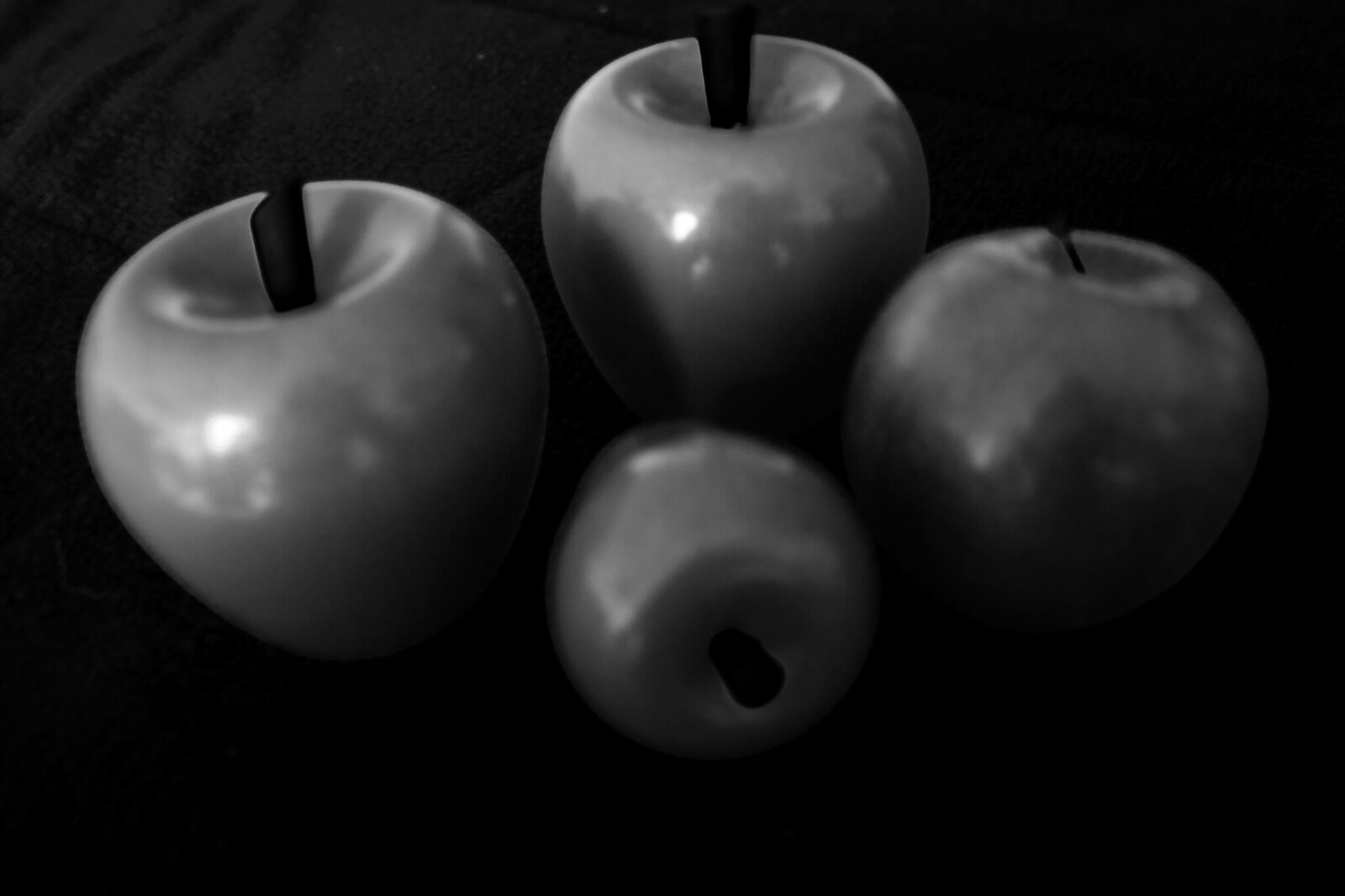In this black-and-white image, four round objects resembling cherries or apples are arranged on a black cloth or blanket. Three of these glossy, silverish-gray objects are upright, with the fourth one slanted on its side. The stems, disproportionately large for three of the objects and small for the fourth, are prominently visible. The three larger objects form a slightly inward-curved row in the background, while the smaller object lies in the foreground with its stem pointing towards the camera. The glossy finish suggests they might be artificial, serving decorative purposes.